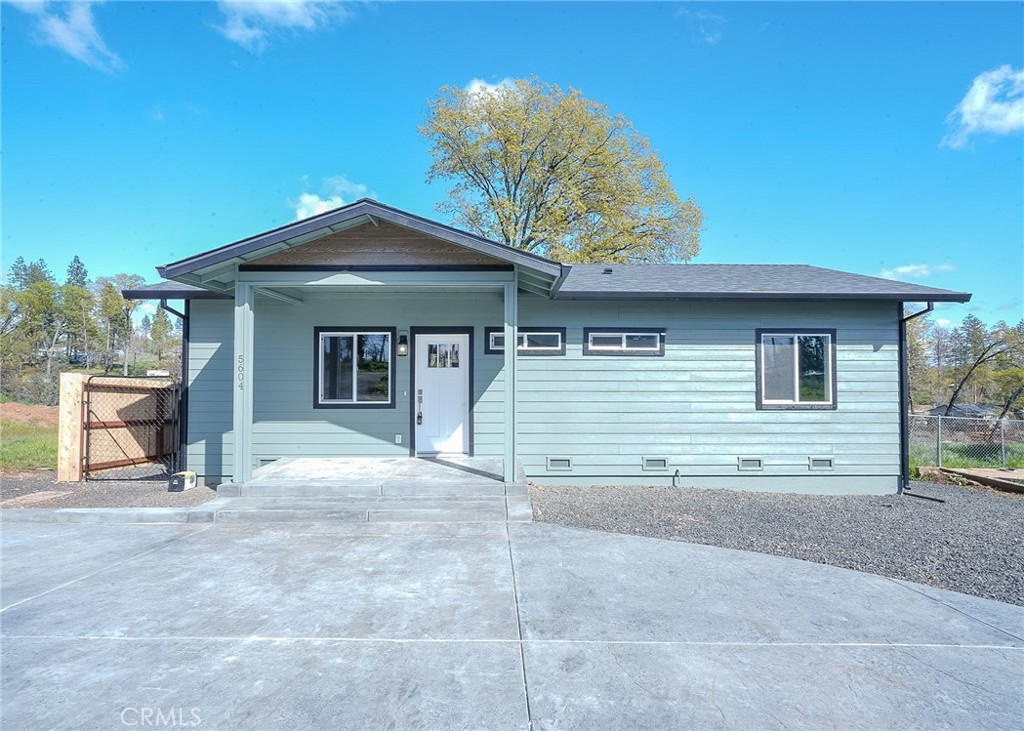This is a horizontal rectangular photograph of a newly constructed, one-story house with a still unoccupied aura. The house, clad in light blue aluminum siding, features a spacious cement driveway at the front, complemented by a patch of gray stone gravel on the right side, which transitions to the back of the property. The entrance area boasts a white front door with three glass panes, sheltered by a wooden canopy supported by sleek, gray metal pillars. The front facade includes a large window to the left of the door and another window on the far right end of the building. Along one side of the house, there are two high-placed windows and an additional window further down, beside which a fence runs parallel to the structure. The yard area exhibits a blend of cement paving and grass, suggesting a rural setting. The overall immaculate appearance, with everything looking shiny and new, underscores that the building has not yet been inhabited, contributing to its austere feel, with no signs of life around it.